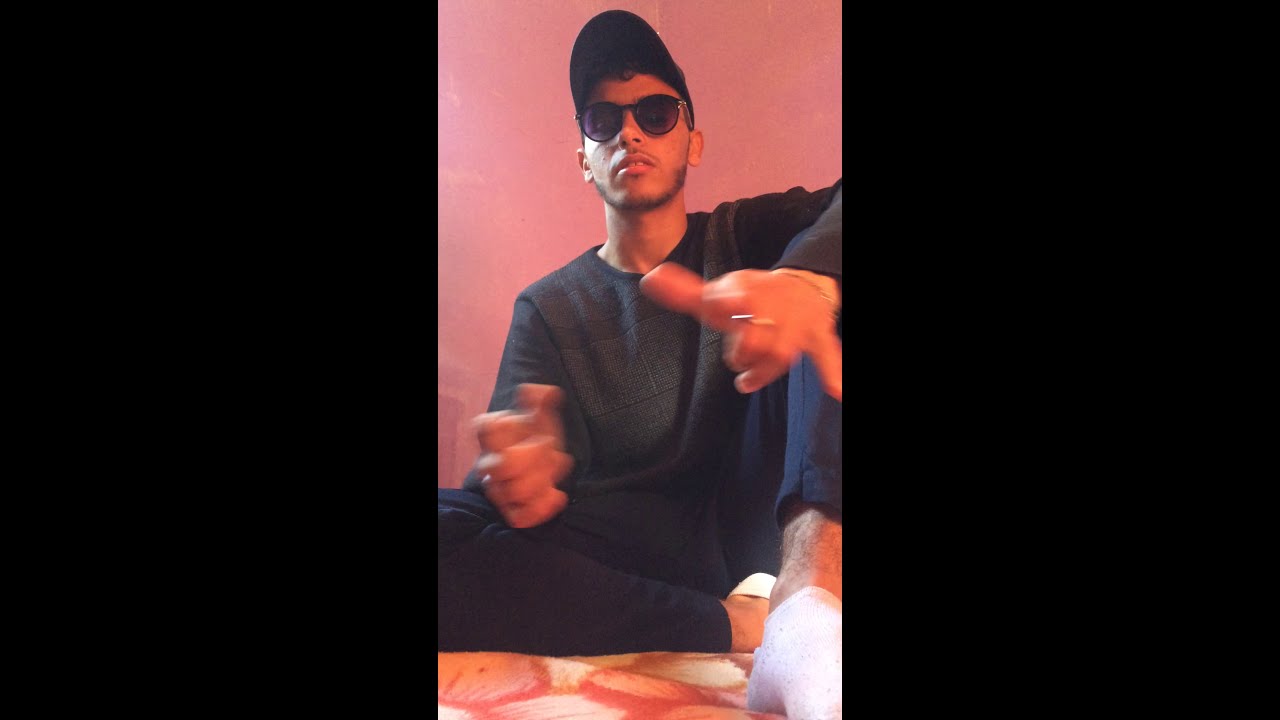This photograph captures a young man sitting on an orange, brown, and white cushion, likely a floral or patterned design. He is dressed in loose, black pants—possibly sweatpants—a black long-sleeve shirt or sweater, and white ankle socks. A slight beard adorns his chin and cheeks, and he sports dark sunglasses along with a black baseball cap positioned at a jaunty angle. His hands are in motion, creating a blurred effect, and he appears to be gesturing. Notably, he wears a ring and possibly a watch. The perspective of the image is level with his feet, looking upward at him as he looks down. The background features a pinkish or coral-colored wall bathed in a bit of natural light. The picture is framed with vertical black borders on the left and right sides.